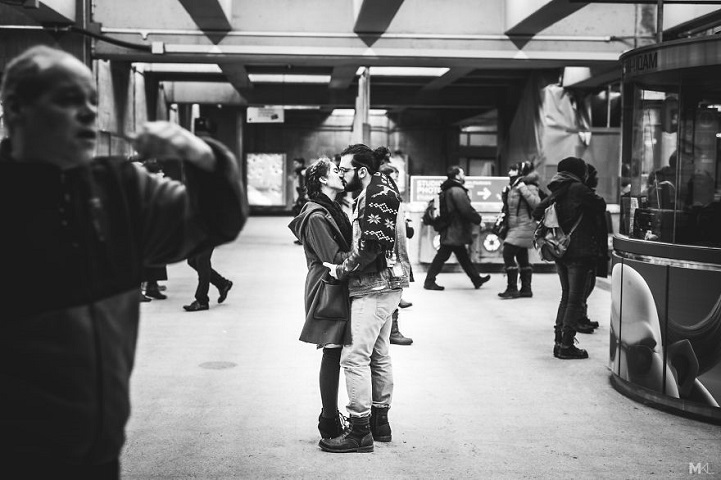This horizontal black-and-white photograph captures an intimate moment in what appears to be a bustling train or subway station, possibly in New York City. Central to the image is a close-up of a couple, a man and a woman, sharing a passionate kiss while hugging each other tightly. The man, with his hair pulled back into a man bun and wearing glasses, is dressed in a sweater featuring an Aztec design, layered with a jean jacket vest, jeans, and boots. The woman, whose hair is styled in braids and pulled back, dons a long wool coat that reaches her legs and either tall boots or lower boots with high socks.

To the right of the couple, a man is seen lifting his head with his left arm raised, possibly to scratch his head or blow his nose. The station is portrayed as a busy place with several people walking to and from different directions. There is also a noticeable booth to the right, likely a place where one might ask for directions or purchase tickets. The scene exudes a cinematic quality, capturing a fleeting, romantic moment amid the everyday hustle and bustle of city life.